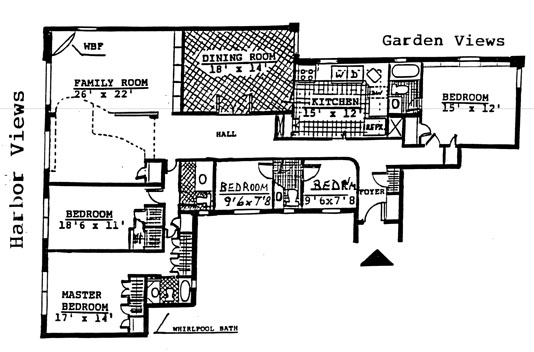This detailed black and white floor plan illustrates a residence labeled "Harbor Views" on the left side. At the top left corner, the family room, measuring 26 by 22 feet, is noted with the initials W, B, F. Adjacent to the family room on the right is the dining room, featuring a crisscross pattern and measuring 18 by 14 feet. Below the dining room runs a hallway. To the right of the dining room lies the kitchen, depicted with a stove, sink, and countertops, marked with a square pattern and measuring 15 by 12 feet.

Adjacent to the kitchen is a bathroom complete with a tub, toilet, and sink. To the right of this bathroom is a bedroom measuring 15 by 12 feet, positioned under the label "Garden Views."

In the lower left portion beneath the family room, another bedroom measures 18 feet 6 inches by 11 feet. Directly below this bedroom is a master bedroom measuring 17 by 14 feet, which includes an adjoining bathroom with a whirlpool tub on the right.

Returning to the center of the floor plan, below the hallway is a compact bedroom measuring 9 by 7 feet 8 inches. To the left and right of this bedroom are additional bathrooms. Finally, the layout concludes with a small bedroom measuring 9 feet 6 inches by 7 feet 8 inches situated at the far right.